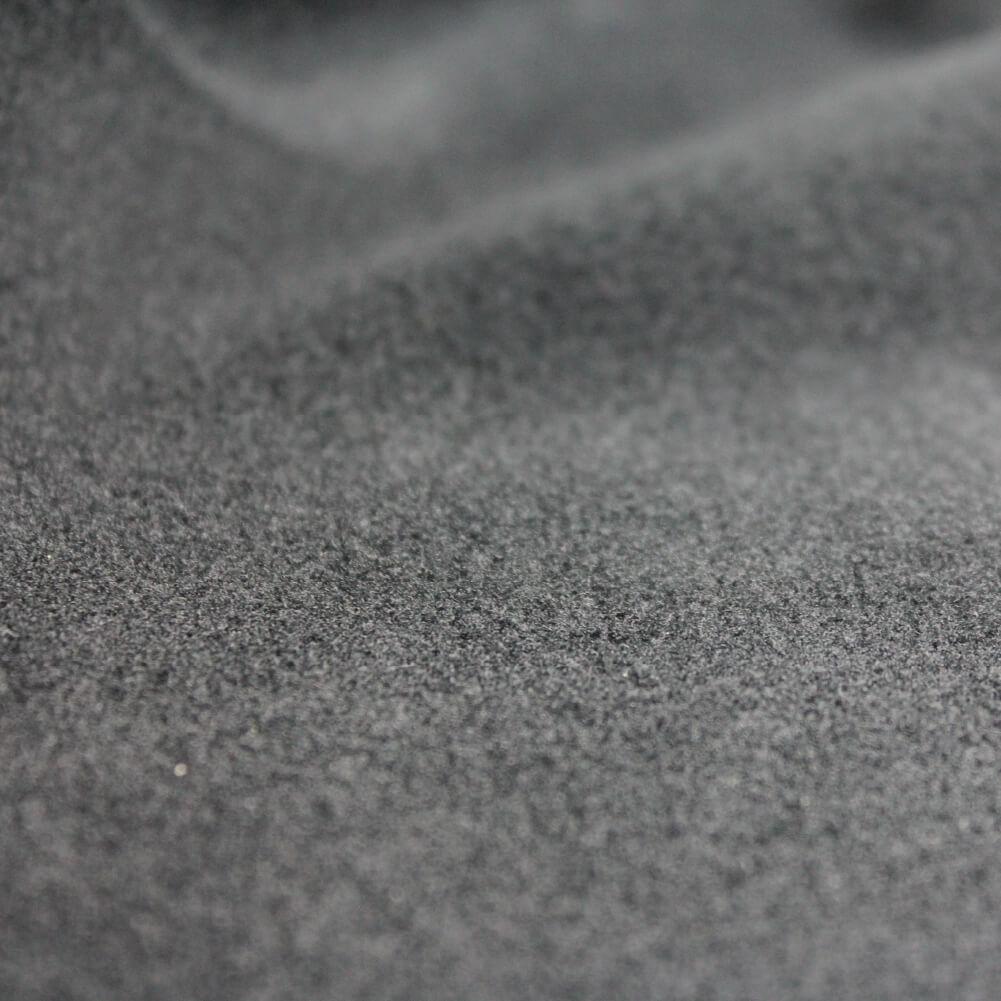The image is a black-and-white close-up photograph capturing a textured surface that appears to be sand or fabric. The photo features coarse grains and tiny pebbles, all in shades of gray, white, and black. The composition reveals a distinct band about one-third to halfway up the image where the individual particles are in sharp focus, allowing you to see the fluffy texture and potential small rocks. The top and bottom portions of the image are notably blurry, possibly due to the texture's curvature or movement, such as wind-blown dust or fabric wrinkles. The entire frame is filled with this material, and no text is present. The detailed focus and quality suggest the use of a macro lens and professional lighting to capture the fine details, making it appear to be either sand with ripple patterns or a fabric with a grainy, fluffy texture.